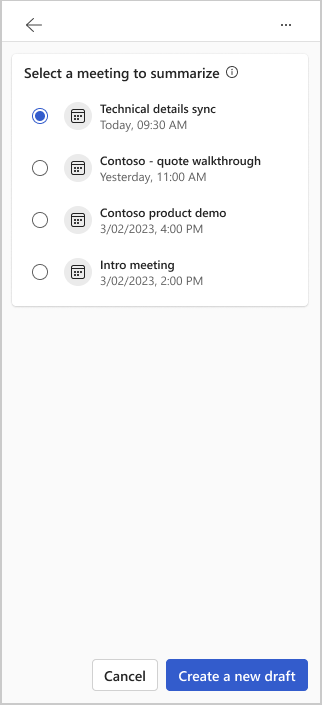This screenshot captures a mobile phone application with a minimalist interface. At the top, a white header spans the width of the screen, featuring a dark grey left-pointing arrow on the far left and three horizontally-aligned dark grey dots on the right. Below the header, a thin, medium grey line separates it from the main body of the page, which has a light grey background.

A prominent white pane occupies about one-third of the page's height, bordered by slightly rounded corners and a thin light grey outline. In the top left corner of this pane, bold text instructs, "Select a meeting to summarize." Adjacent to this text, towards the right, is a dark grey eye icon enclosed in a dark grey circle.

Underneath this header, there are four radio buttons, each accompanied by relevant information. The first radio button is a blue circle with a white outline and a thin blue border. Next to it is a light grey circle containing a dark grey calendar icon. To the right, the first meeting is labeled in bold dark grey text as "Technical Details Sync," with the subtext in light grey noting, "Today, 9:30 AM." 

The remaining radio buttons, distinguished by white circles with thin dark grey outlines, follow a similar layout:
- The second radio button corresponds to "Contoso-Quote Walkthrough," tagged with the subtext "Yesterday, 11:00 AM."
- The third is labeled "Contoso Product Demo," scheduled for "3-02-2023, 4:00 PM."
- The last button indicates "Intro Meeting," also set for "3-02-2023," but at "2:00 PM."

The bottom section of the page features a significant expanse of negative space, culminating in two buttons aligned at the bottom. The right-aligned button is wide and blue, with white text stating "Create a New Draft." To its left, a smaller white button with a medium grey outline and grey text reads "Cancel."